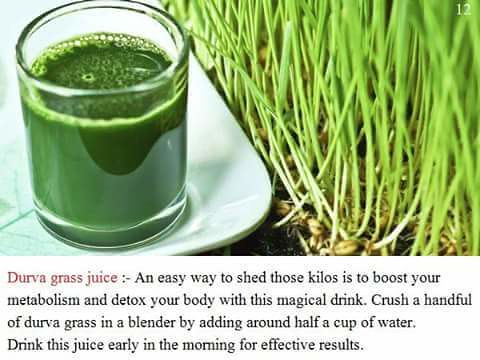This photograph showcases a refreshing green beverage, possibly a green smoothie, served in a clear glass which is neatly placed on a rectangular white plate. Adjacent to the plate and glass is a fresh bunch of Darva grass, adding a natural element to the composition. The text below the image reads, "Darva Grass Juice: An easy way to shed those kilos is to boost your metabolism and detox your body with this magical drink. Crush a handful of Darva grass into a blender by adding around half a cup of water. Drink this juice early in the morning for effective results." The image and accompanying text suggest a healthy, natural approach to weight loss and wellness through the consumption of Darva Grass Juice.